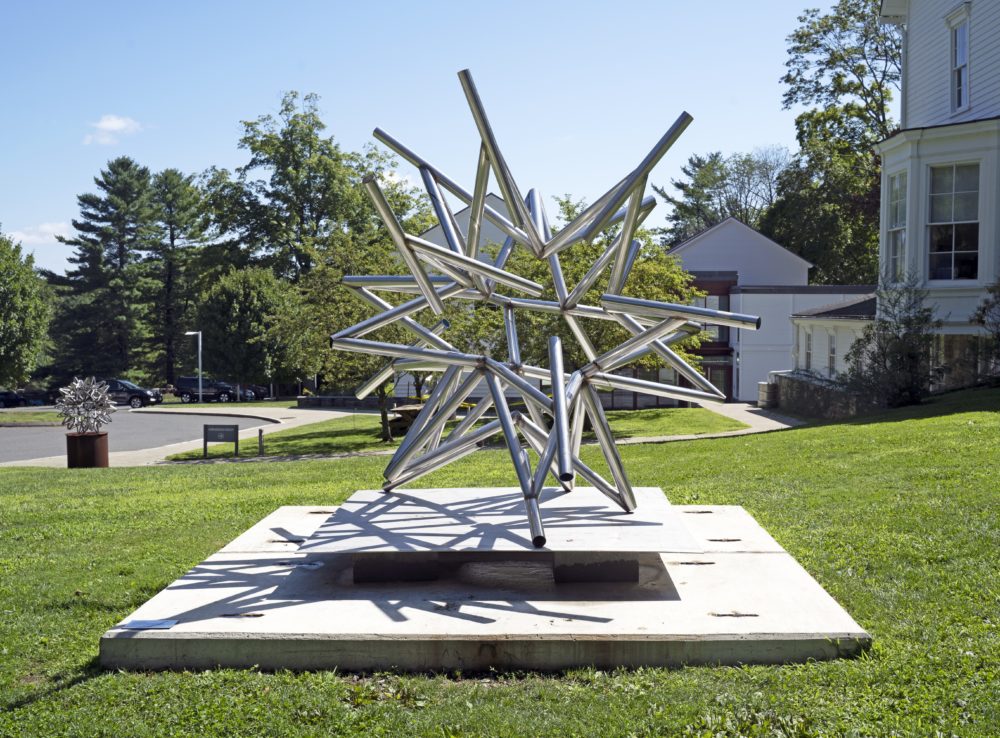This color photograph was taken on a bright sunny day with a clear blue sky and only a few scattered clouds. The scene is set on a vibrant green lawn, showcasing a modern art sculpture in the center. The sculpture, crafted from silver metal tubes, forms an intricate, star-like structure with numerous spiky projections. It stands atop a two-stepped, white concrete pedestal; the lower platform is larger with a smaller raised platform directly beneath the sculpture. Surrounding the sculpture are various buildings, including white clapboard houses visible on the right side of the image. On the left, there is a road and a brown pot containing a smaller, similar metallic sculpture. In the background, a wooded area with several pine trees can be seen, adding to the scenic backdrop. There are also a few vehicles parked, suggesting the presence of a nearby parking lot. Notably, the photograph contains no people or animals.